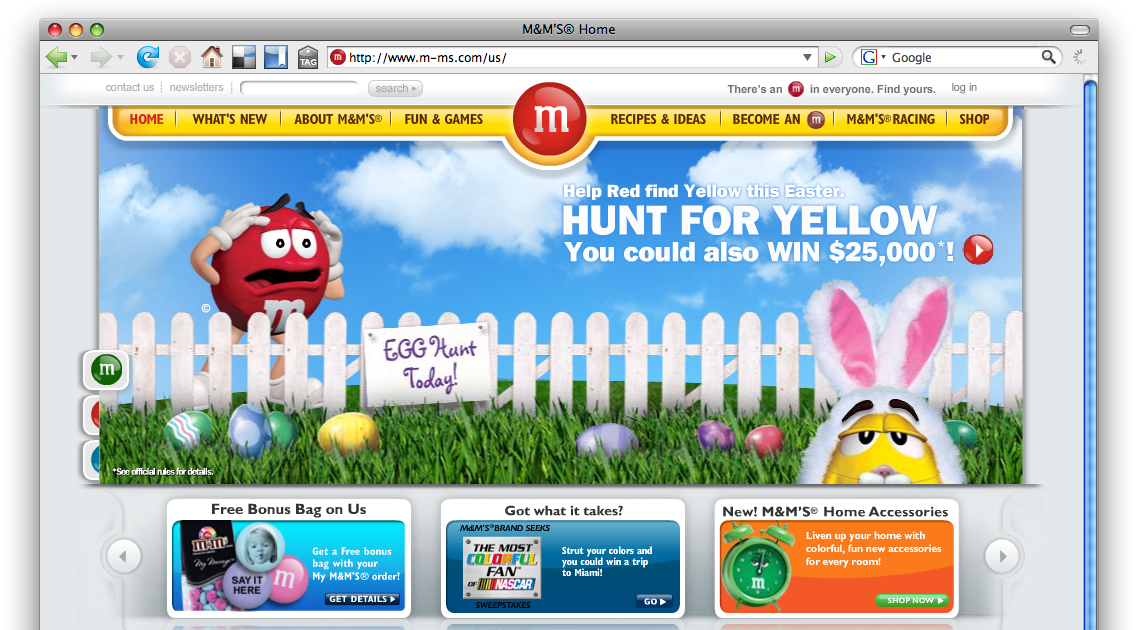On a computer screen, the search bar at the top displays "M&M's home." The main image on the screen depicts a charming Easter scene with a long white picket fence, lush tall green grass, and colorful pastel Easter eggs scattered throughout. The eggs are painted in soft blues, greens, yellows, and pinks, adding to the festive atmosphere.

Front and center, a familiar M&M's character appears—this time, the red M&M, looking distressed. His eyebrows are raised in worry, his mouth slightly open, and his white-gloved hands rest on top of his head. To the right corner, another M&M character makes an appearance—the yellow M&M, humorously dressed in a full bunny suit, complete with tall pink ears.

The screen displays an enticing message in white text: "Help find Yellow this Easter. Hunt for Yellow." It further teases, "You could win $25,000!" There is a red circle featuring a lowercase 'm' at the top, representing the M&M candy brand.

Additionally, several navigation options are visible, including "Home," "What's new about M&M's," "Fun and Games," "Recipes and Ideas," "Become an Insider," "M&M's Racing," and "Shop," inviting users to explore more about M&M's.